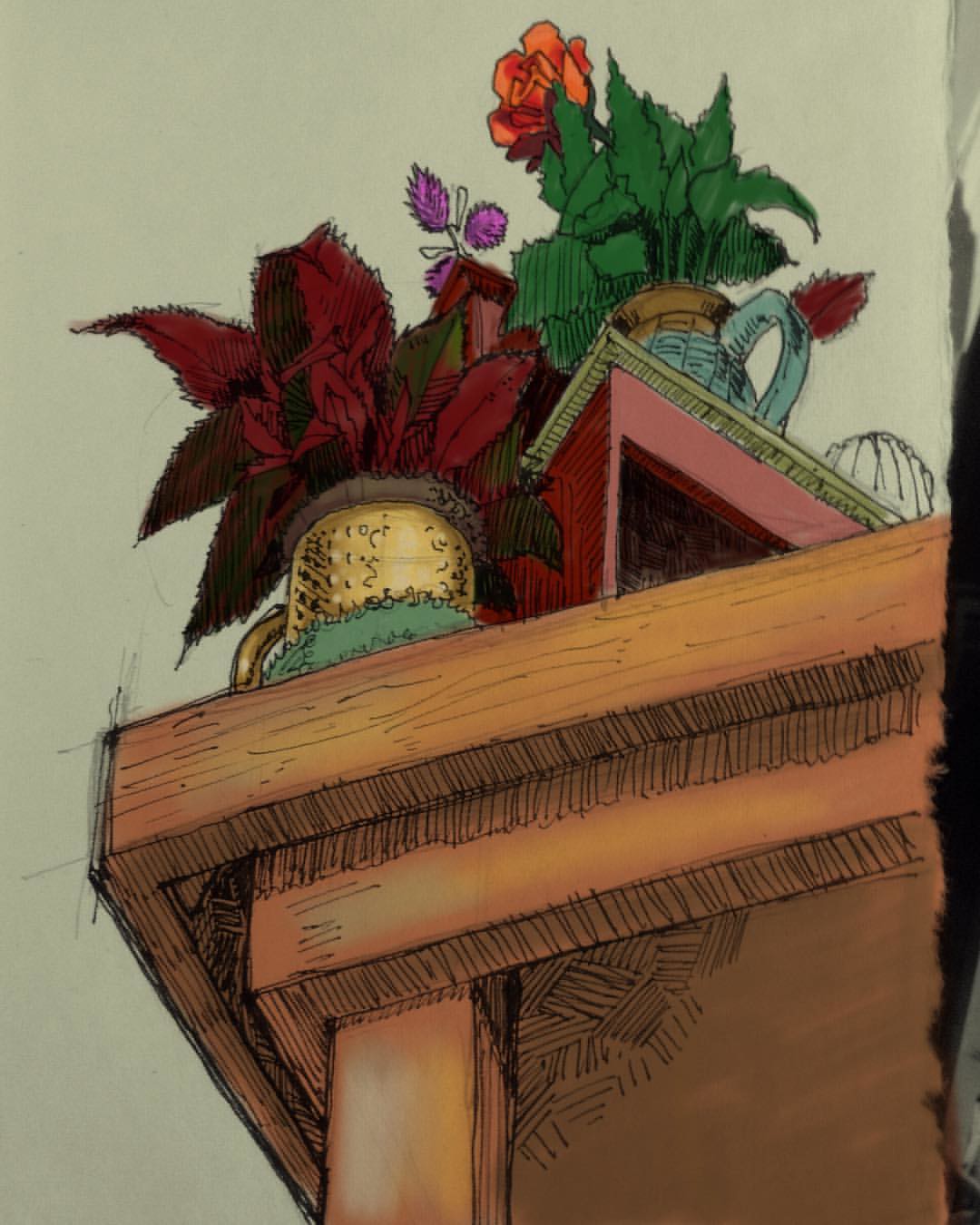The image depicts a detailed artist's drawing viewed from a low perspective, looking upwards at a corner of a brown wooden table set against a grayish background. The table's construction is visible, including a 4x4 wooden post supporting it, with multiple 2x6s nailed on the sides and spacers in between. Atop the table, there is a golden mug with a handle on the left, containing dark red poinsettia-like leaves accented with green at the base. To the right of this mug, a box-like structure supports a teapot-shaped pot that is light blue with spiral black lines and a light brown rim. This pot holds an orange rose and long green leaves. Pencil marks detail the edges and emphasize the artistic nature of the depiction.